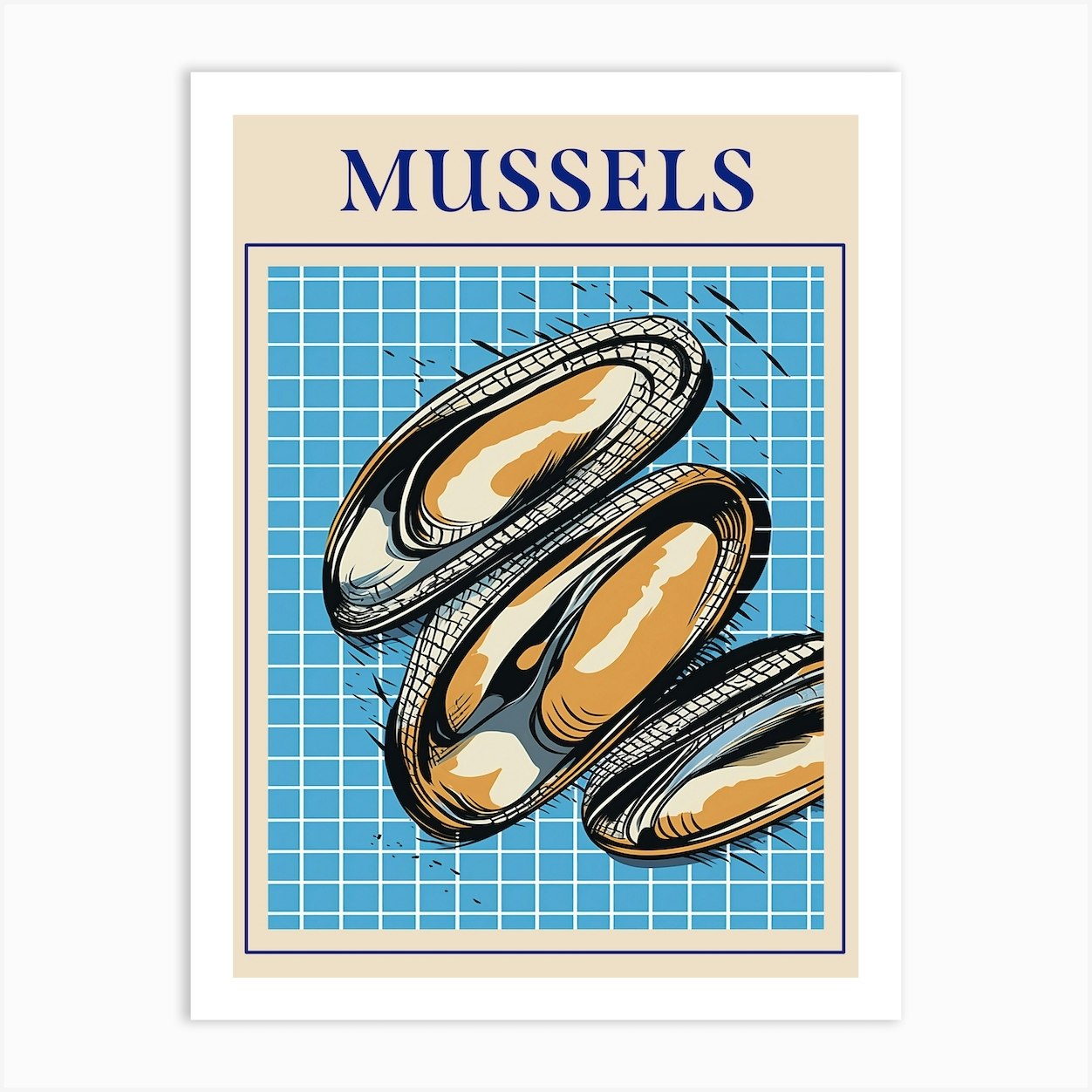This is a poster, bordered in white, featuring a pinkish background. At the top, "Mussels" is prominently written in navy blue letters. The poster showcases a detailed illustration of three mussels, each one open, with black shells and interiors shaded in tan and white. These illustrations rest on a blue background, which is patterned with a white grid creating square boxes. The mussels are meticulously drawn, capturing their texture and colors, making the image appear almost like a cover illustration for a seafood magazine.